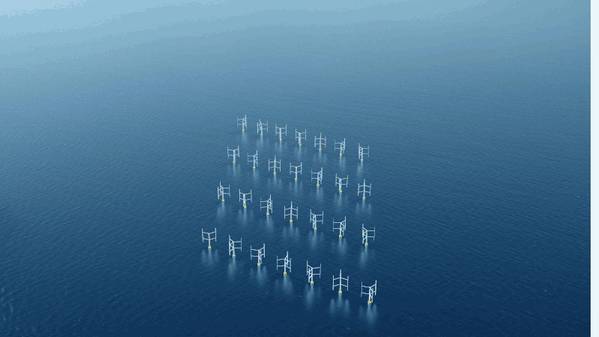In this aerial view, 28 wind turbines are installed in the middle of a vast body of water, likely at sea or in a large lake. The turbines are arranged in four distinct rows of seven, totaling 28 individual units. Each turbine features three blades mounted on top of the generator. There is no text in the image, and apart from the wind turbines, the rest of the scene is dominated by the expansive blue water. The turbines appear to be stationary, with their blades aligned consistently, pointing downward towards the bottom of the image. The photograph, captured from a significant height, possibly by a drone or helicopter during daylight, focuses solely on the wind turbines without revealing any other landmarks or signs of location.